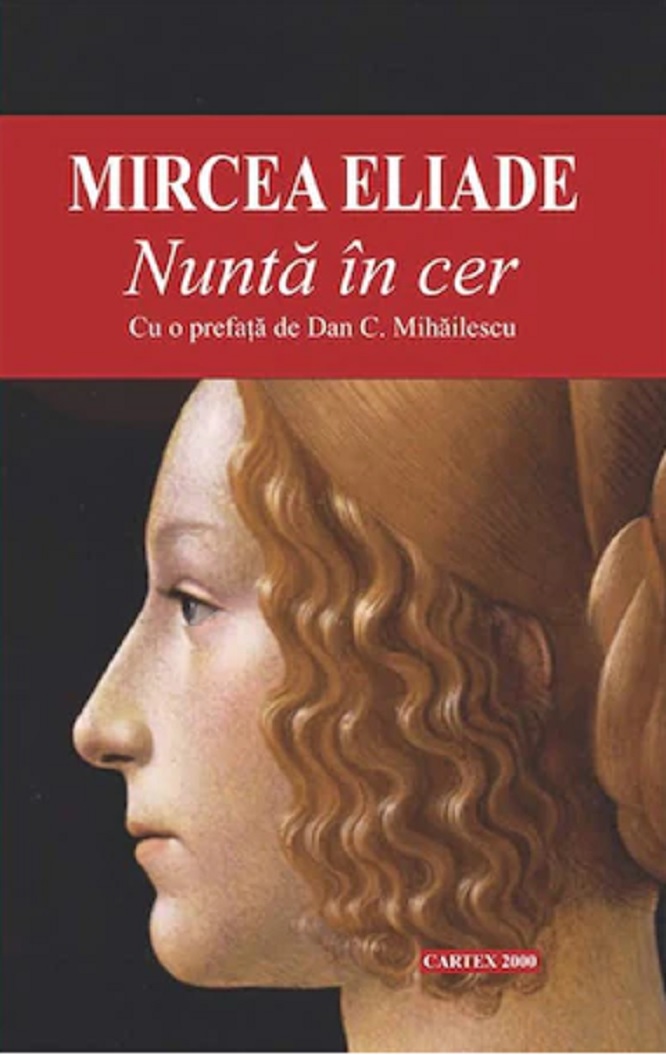The book cover features a detailed and elegant design. Dominating the cover is an artistic side profile of a young white woman with classic beauty, her blue-green eyes gazing to the left. She has reddish-blonde hair styled in a bun, with soft curls subtly framing her slender face. The background is a stark black, accentuating the refined features of the woman.

The title of the book, "Mircea Eliade Nunta in Ser," is prominently displayed across a striking red banner at the top of the cover, in white serif text. "Mircea Eliade" is in all caps, while "Nunta in Ser" is in italics, except for the capitalized initial letters. Below the title, in a smaller, non-italicized font, reads "Cuo Prefata de Danci Mihaliescu," indicating additional content or contributions by another author.

Near the bottom right of the cover, another red rectangle holds the text "CARTEX 2000," also in white all caps, providing a uniform and cohesive design element that ties the cover together.